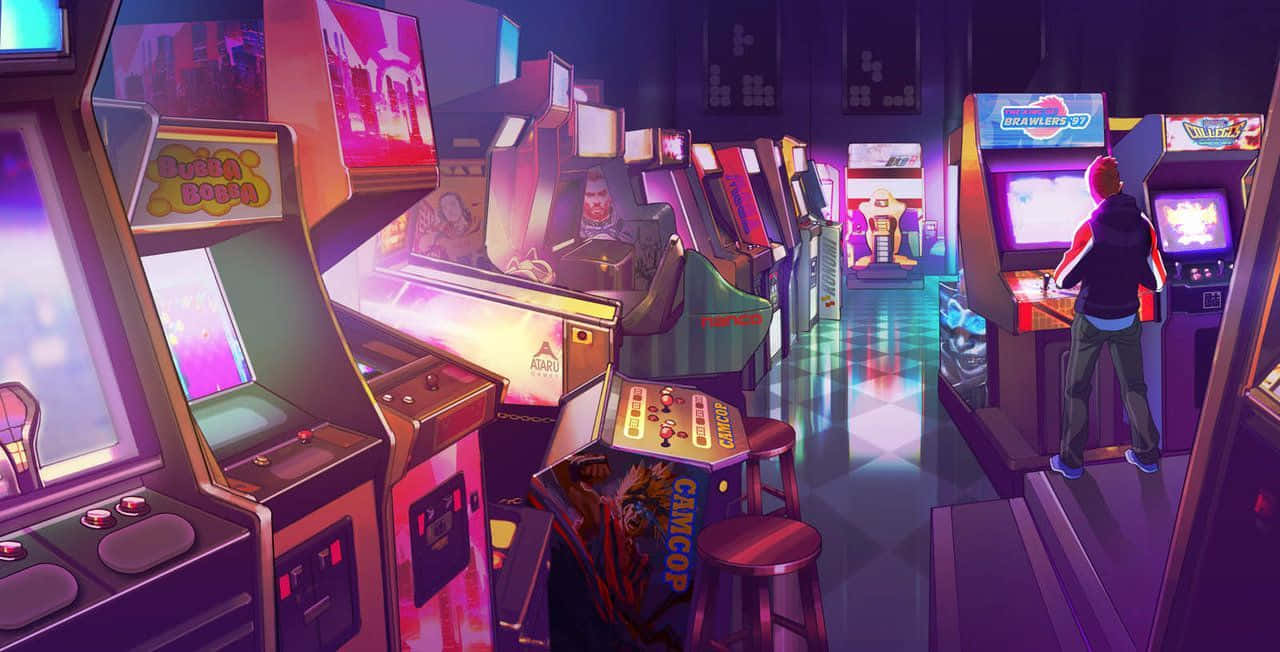The image is a detailed, digital illustration of a nostalgic arcade scene set in a dark room illuminated by the vivid neon lights of numerous closely-packed, old-style arcade machines. A young male, positioned on the right side of the image, is engaged in playing a game titled "Brawlers 97." The boy is viewed from behind and is dressed in a black hoodie accented with red, white, and black vertical stripes running down the sleeves. Beneath the hoodie, a glimpse of his blue t-shirt is visible, and he pairs his outfit with gray jeans or sweatpants and blue tennis shoes. The arcade is filled with a variety of labeled machines including "colleges," "Bubba Bubba," "camcop," "Itaru," "Nanko," and "Konomi." The setting features a black and white checkered linoleum floor reminiscent of the 80s, with light from the game screens reflecting off it. Scattered stools and stylized background images of Tetris add to the authentic retro arcade atmosphere.